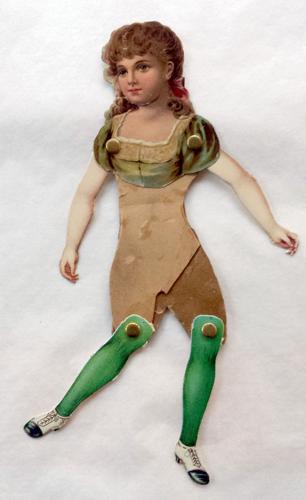The image depicts an old-style paper doll of a young girl, posed against a white background. The doll is articulated with gold brads, allowing movement in her limbs. She has long, curly orange hair with bangs that cascade down her back. Dressed in a brown outfit, she features intricate green shoulder decorations. From the knees down, she is adorned in green stockings and wears white shoes with black tips. Her arms, which do not match the color of her body, are extended slightly outward, and they are also jointed with brads for mobility. Notably, her left leg juts out crookedly to the side, emphasizing the doll’s charming, handmade nature.